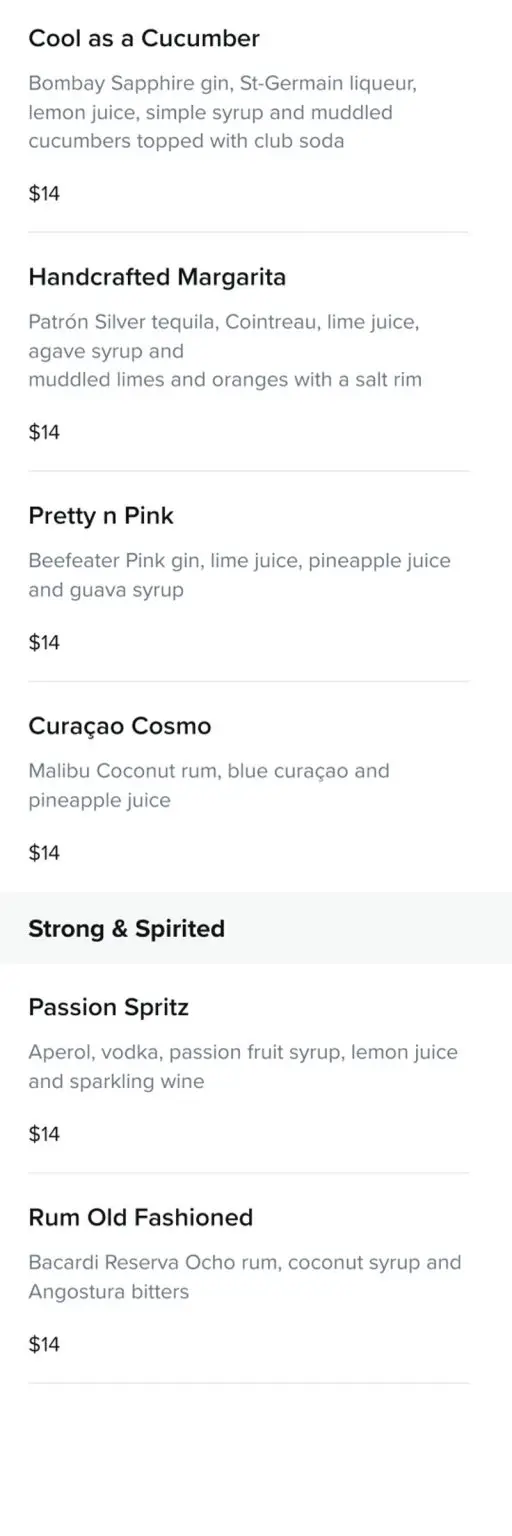The image displays a drink menu on a white background with black text. At the top, it features a section titled "Cool as Cucumber," listing a cocktail made with Bombay Sapphire Gin, St. Germain Liqueur, lemon juice, simple syrup, and muddled cucumber, topped with club soda, priced at $14. Next, it highlights the "Handcrafted Margarita," crafted with Patrón Silver Tequila, Cointreau, lime juice, muddled limes, and orange, served with a salt rim, also priced at $14.

Following that, the menu introduces the "Pretty and Pink" cocktail, which includes Beefeater Pink Gin, lime juice, pineapple juice, and guava syrup, priced at $14. The "Curacao Cosmo" features Malibu Coconut Rum, Blue Curaçao, and pineapple juice, again priced at $14.

Another section titled "Strong and Spirited" details the "Passion Spirits" cocktail, which combines Aperol, vodka, passion fruit syrup, lemon juice, and sparkling wine, priced at $14. Finally, the "Rum Old Fashioned" is described, made with Bacardi Reserva Ocho Rum, coconut syrup, and Angostura bitters, also priced at $14.

In summary, the menu highlights a variety of handcrafted cocktails, each priced at $14.